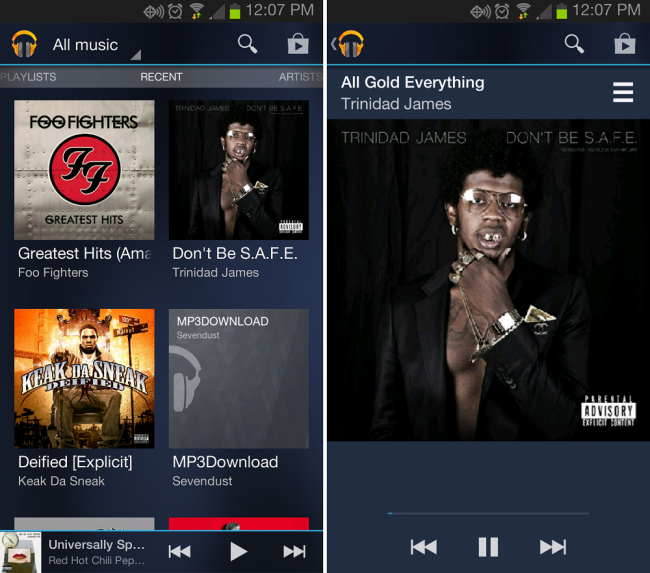This image features two adjacent smartphone screenshots presented in a portrait orientation, separated by a thin white border. Together, these two screenshots form a nearly square composition. 

The left screenshot displays a music library interface. At the top, a black bar features an assortment of status icons: a clock reading 12:07 p.m., Wi-Fi signal indicators with a green up arrow and an orange down arrow, a nearly depleted network connection icon, and a vertical battery icon with a green meter. Below this black bar is a header with a headphones logo labeled "All Music," accompanied by a clickable arrow for sorting, a search icon, and a shopping icon. A gray navigation bar underneath offers options for "Playlist," "Recent," and "Artists." Below the navigation bar, there are four album thumbnails: "Greatest Hits" by Foo Fighters, "Don't Be S.A.F.E." by Trinidad James, "Deified" by Keak Da Sneak, and "MP3 Download" by Sevendust.

The right screenshot shows the playback screen for the selected track "All Gold Everything" by Trinidad James. It shares the same black status bar at the top. Below this, a header features an image of Trinidad James facing the viewer, with a hamburger menu icon on the top right. The playback interface displays the track's title, a progress bar indicating that the track has just begun, and control buttons for reversing, fast-forwarding, and pausing.